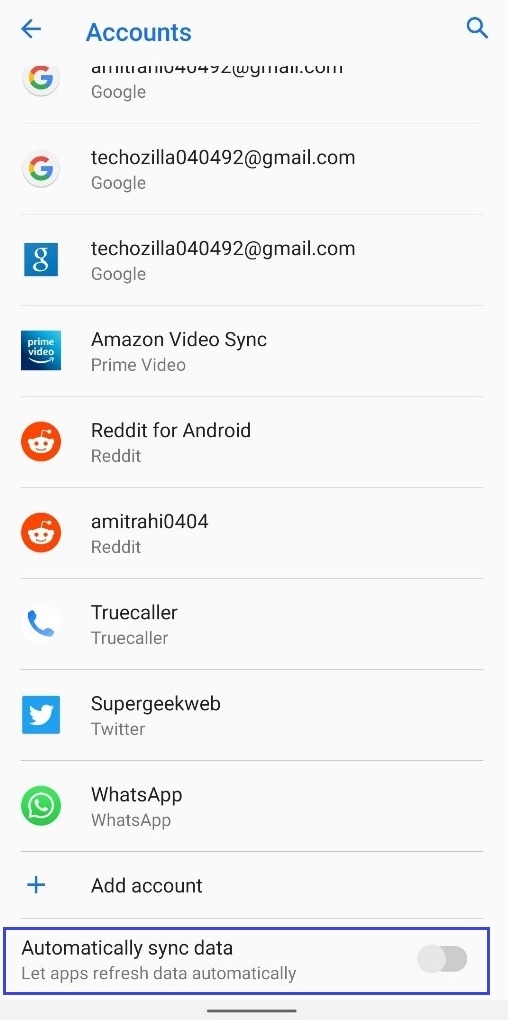The image depicts the Account Settings page of an Android phone, showcasing a variety of linked accounts and their synchronization settings. The page is organized with a list of accounts, including:

1. **Google Account:** tekuzilla0404492@gmail.com
2. **Amazon Video Sync**
3. **Reddit for Android**
4. **Truecaller:** amitavv0404
5. **Twitter:** supergeekweb
6. **WhatsApp**

Each account is listed with corresponding synchronization options. A highlighted section in purple emphasizes the "Automatically sync data" setting, which allows apps to refresh their information automatically. Next to this text is a toggle switch, providing an option to enable or disable this sync feature.

At the top of the page, in the center, is the title "Accounts" indicating the current settings being viewed. The top-left corner features a back icon for returning to the previous screen, while the top-right corner houses a search icon, allowing for easy navigation and account search capabilities within the settings page.